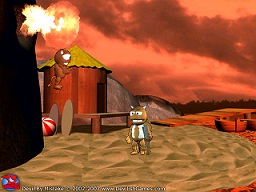The image depicts a low-resolution character design from an older video game, featuring a vibrant, geometric setting. The backdrop showcases a detailed sky, strikingly reminiscent of a wildfire, painted in intense hues of orange and red, with cloudy textures. Trees and mountains are visible in the distance, adding depth to the scene. In the foreground, a sandy terrain extends across the base, where a small beach hut with an orange facade and yellow roof stands. This hut is accompanied by surfboards and a red and white striped beach ball.

The scene is populated by two cartoonish creatures resembling chipmunks or beavers, distinguished by their exaggerated features — white eyes, white mouths, and white ears but notably lacking noses. One character hovers mid-air, seemingly suspended above the sandy ground, while the other, donning a shirt and tie, walks below. The floating character has flame-like elements above its head, adding to the dramatic ambiance.

A brown wooden dock and a boat are situated near the hut, enhancing the coastal vibe. Despite the geometric simplicity of the sand, its texture remains impressively high-quality. The bottom corner of the photo contains illegible text, likely credits, but the small size of the image makes it difficult to discern.